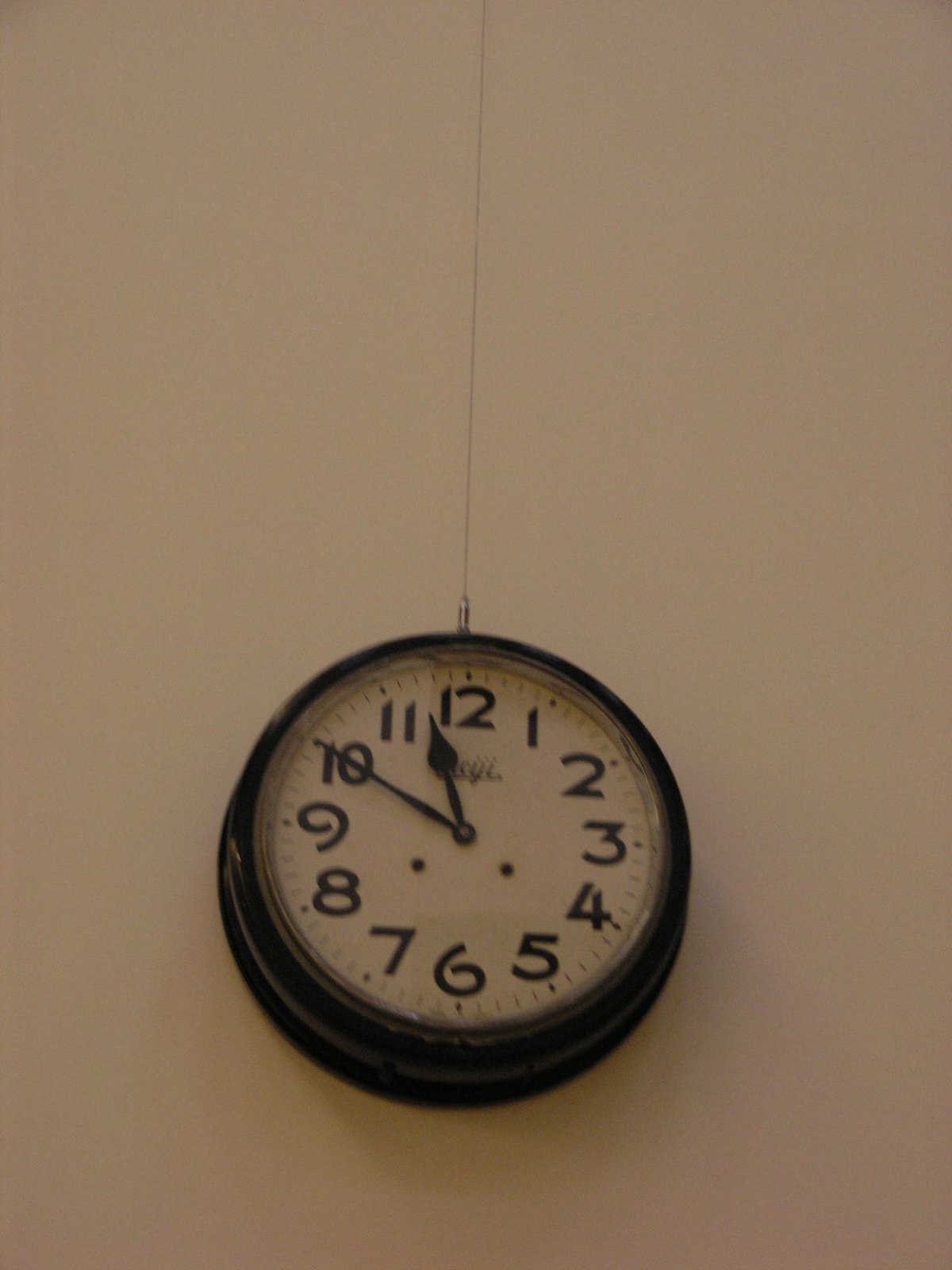The image captures an upward view of a hanging clock. The clock is suspended by a single, thin wire that descends significantly from an unseen attachment point above. The clock itself is circular with a sleek black outer rim and a contrasting white face. Prominently displayed on the face are black numerals arranged in a typical clock pattern: starting at 12 at the top, followed by 1, 2, and 3 on the right, descending to 4, 5, and 6 at the bottom, then ascending from 7, 8, and 9 on the left, and finally reaching back up to 10 and 11 before returning to 12. The clock's hands are also black, with the long minute hand pointing at the 10 and the shorter hour hand positioned between the 11 and 12. Below the clock hands are two small black dots. The background is a light brownish-gray wall, providing a muted backdrop that makes the clock stand out prominently.